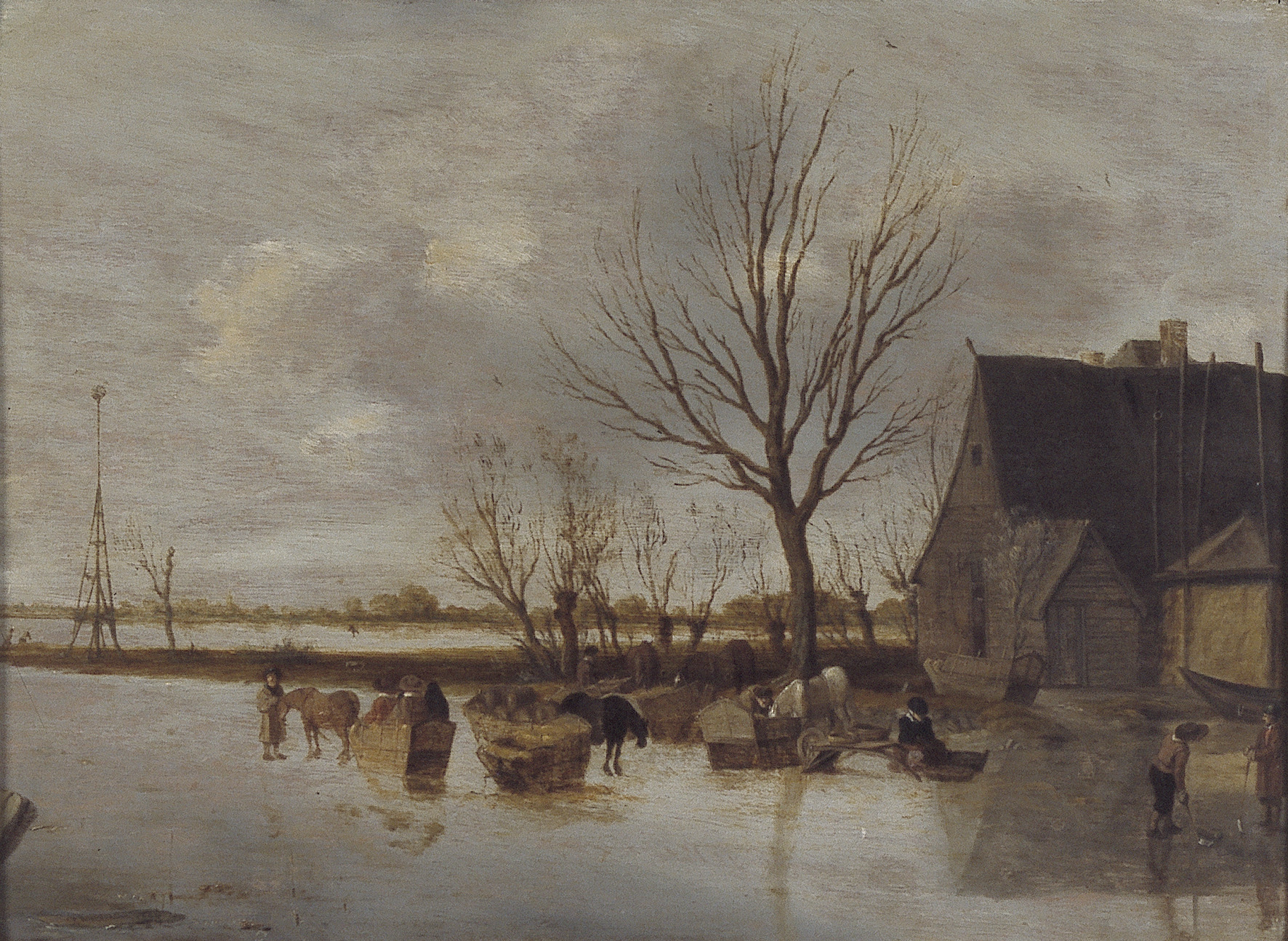The painting depicts a bleak, monochromatic outdoor scene characterized by muted grays and sepia tones. The sky is a foreboding mix of browns and grays, evoking a sense of dreariness. Central to the composition is a large, nearly barren tree with sparse branches, surrounded by smaller leafless trees. In the middle ground, a group of horses stands in what appears to be water or wet ground, possibly a wetland area. Adding to the rustic atmosphere, a bale of hay and a horse-drawn wagon with a man standing beside it are prominently featured. To the right, a ramshackle house with a darker brown roof stands, with two people conversing nearby. Further enhancing the sense of desolation, a windmill and a distant row of trees are visible on the horizon, framed by a gray and cloudy sky.